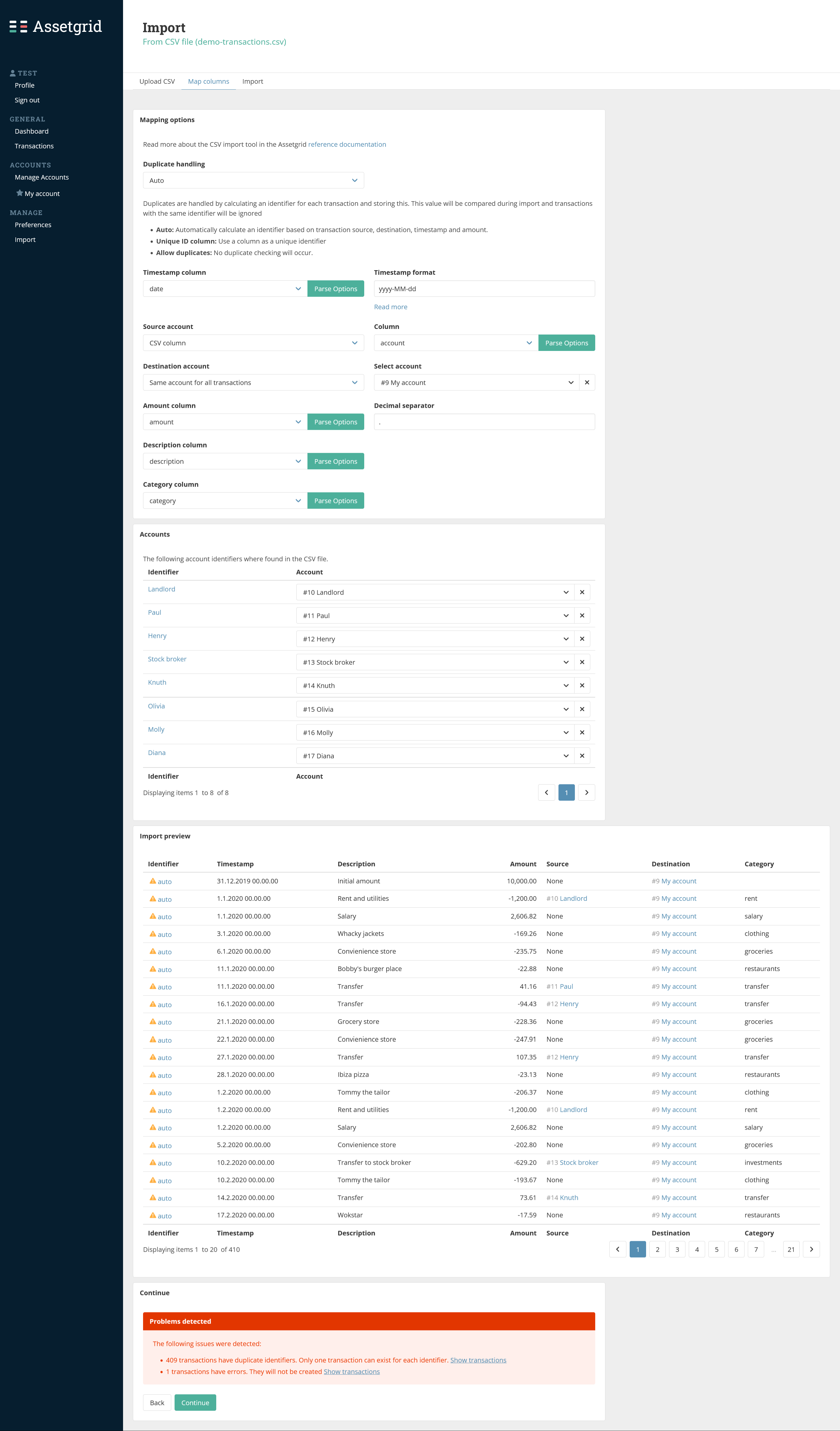This image depicts a detailed snapshot of a computer screen or web page featuring a vertically oriented layout. On the left side, a dark vertical column, around one-seventh of the total width, serves as the menu bar. The menu bar is labeled "Assignment" and comprises at least 10 sub-items, though the text is not legible due to the extensive zooming.

On the right-hand side, the word "Export" is prominently displayed, accompanied by several clickable elements. Dominating approximately 90% of the screen is a large gray box filled with intricate details that are challenging to discern. At the top of the screen, clickable items are bordered in green, but their titles remain unreadable.

The middle section features multiple blue-titled items, which likely indicate clickable links with dropdown arrows for additional information. The lower portion of the image contains about 15 rows. The first row appears to represent a folder, while the subsequent rows, possibly indicating phone numbers, are exceedingly small and difficult to decipher.

At the very bottom is a red box, which traditionally signifies a warning or important note, typically about maintaining the integrity of the assignment. Overall, the text throughout the image is minutely detailed, making it extremely hard to read.